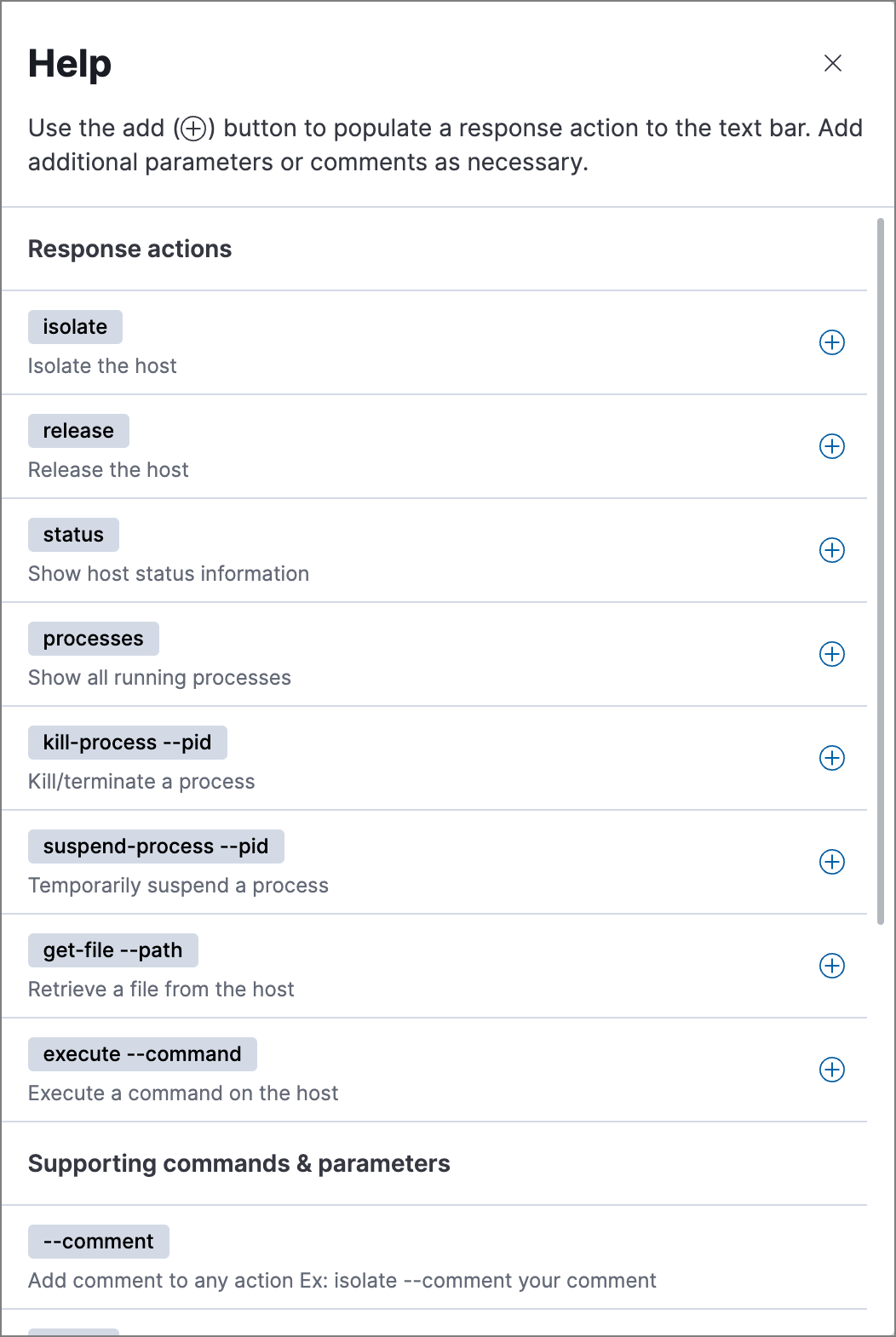**Screenshot Description: Detailed Interface Guide**

This screenshot captures a section of a user interface. 

- At the top left corner, the word "HELP" is prominently displayed in large, bold black letters.
- In the top right corner, there is a small "X" button.
- Beneath "HELP," there is an instructional text which reads: "Use the add (+) button to populate a response action to the text bar, add additional parameters or comments as necessary."
- Below this instructional text, a header titled "Response Actions" is displayed.
- Under the "Response Actions" header, there is a list of actions, each highlighted in a grey box. Each action is followed by descriptive text:
  - **Isolate:** Isolate the host.
  - **Release:** Release the host status.
  - **Show Host Status:** Show host status information.
  - **Processes:** Show all running processes.
  - **Kill Process (PID):** Kill/terminate a process.
  - **Suspend Process (PID):** Temporarily suspend a process.
  
- On the right side of the interface, next to each action, there is a circular button with a plus "+" sign inside it, allowing users to add the corresponding action.